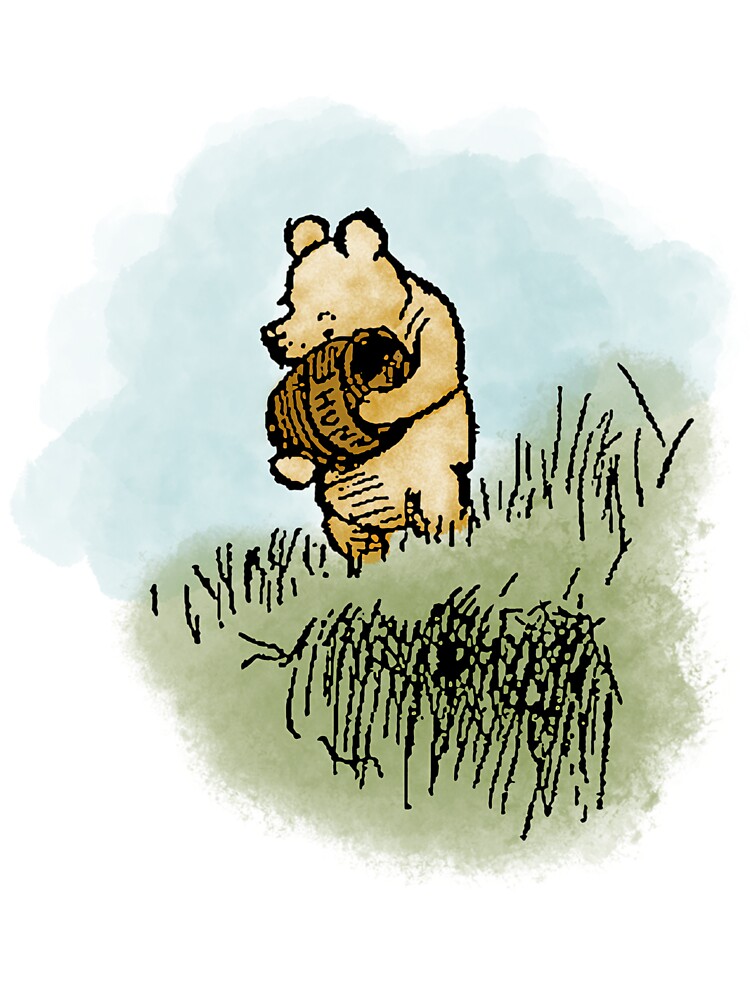This is a charming illustration of Winnie the Pooh, depicted in a simple yet endearing style. Pooh, colored a light tan, is tenderly hugging a barrel of honey labeled "H-U-N-Y." He stands in a grassy area where the tall grass comes up to his ankles, rendered with black lines and a watercolor wash of green, giving it a soft, blurred appearance without distinct edges. Pooh’s head is touching the honey jar, accentuating his fondness for it. The background is a clear blue sky, adding to the serene and joyful ambiance of the scene. The image captures Pooh holding onto his beloved honey with both arms, showing him from a side view as he strolls along the grassy field. It's a very cute and heartwarming portrayal of Pooh, celebrating his simple pleasures.